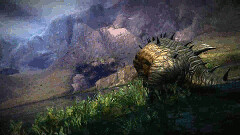The image depicts a scene that is somewhat challenging to decipher. The upper half of the picture transitions from lighter to darker shades of blue as it moves to the right, suggesting perhaps a sky at dusk or an abstract backdrop. Below, the bottom half features a gradient of green, darkening towards the bottom right, which could represent grassy terrain or another abstract layer.

Dominating the right-hand side of the picture is an enigmatic creature that bears semblance to an armadillo or hedgehog in shape. This creature exhibits a distinctive hump along its back, extending into a long tail adorned with black, menacing spikes. The spikes vary in length; those on the uppermost part of the creature are shorter, gradually lengthening as they extend down towards the tip of the tail. The creature's body is distinctly two-toned: the rear half boasts a greenish hue, while the front shifts from yellow to a brownish tint, creating an intriguing contrast. This peculiar coloration and form imbue the creature with an almost mythical appearance.